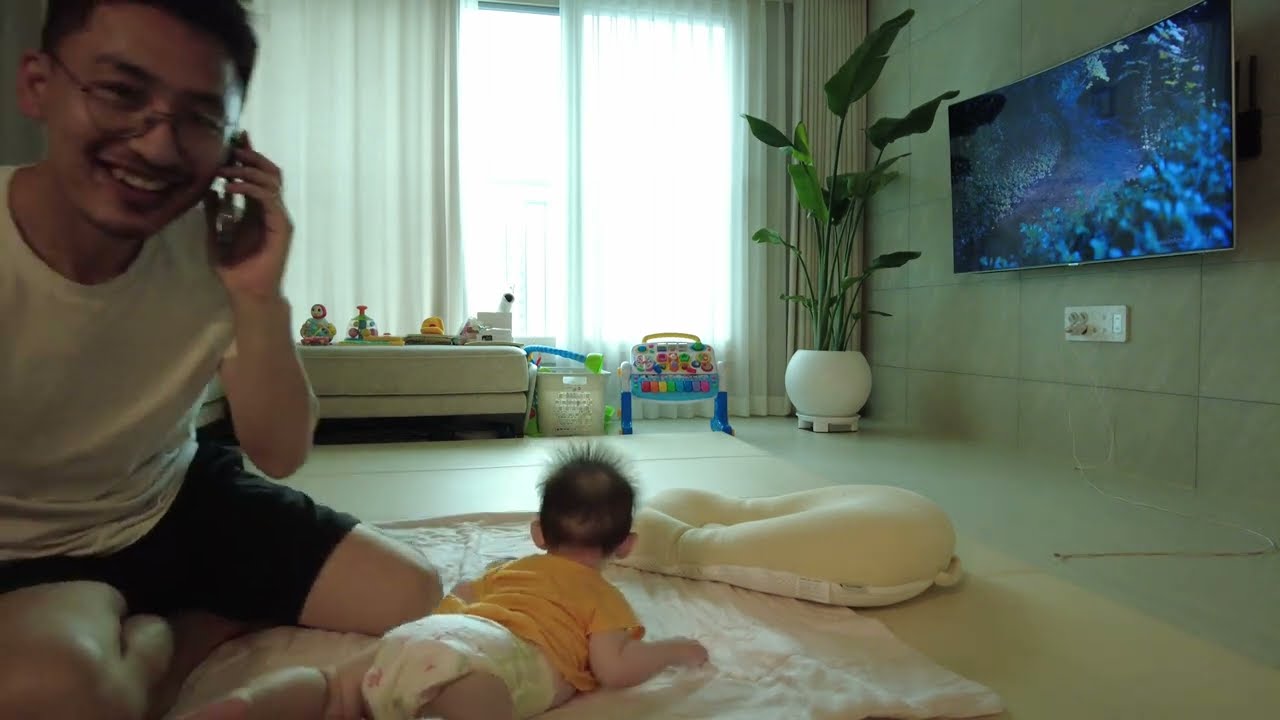In this picture, a young Asian man, probably in his early to mid-twenties, dressed in a white t-shirt and black shorts, is kneeling on a blanket on the floor. He is smiling broadly, holding a phone up to his ear, and wearing glasses. Beside him, a baby with spiky black hair and some bald spots is lying on a mat, facing diagonally from the lower left corner towards the middle of the picture. The baby is propped up on their elbows, wearing a mustard yellow shirt and a diaper with designs. In front of the baby, there is a small cushion, possibly for the baby to rest on. The room has a mix of features, including a tannish-colored tile wall on the right, a large flat screen TV mounted on the wall with a blue aquarium scene displayed, and white curtains covering a big window in the background. Surrounding the area are various baby toys, and there is a tall potted plant, about six feet tall, positioned to the left of the TV.